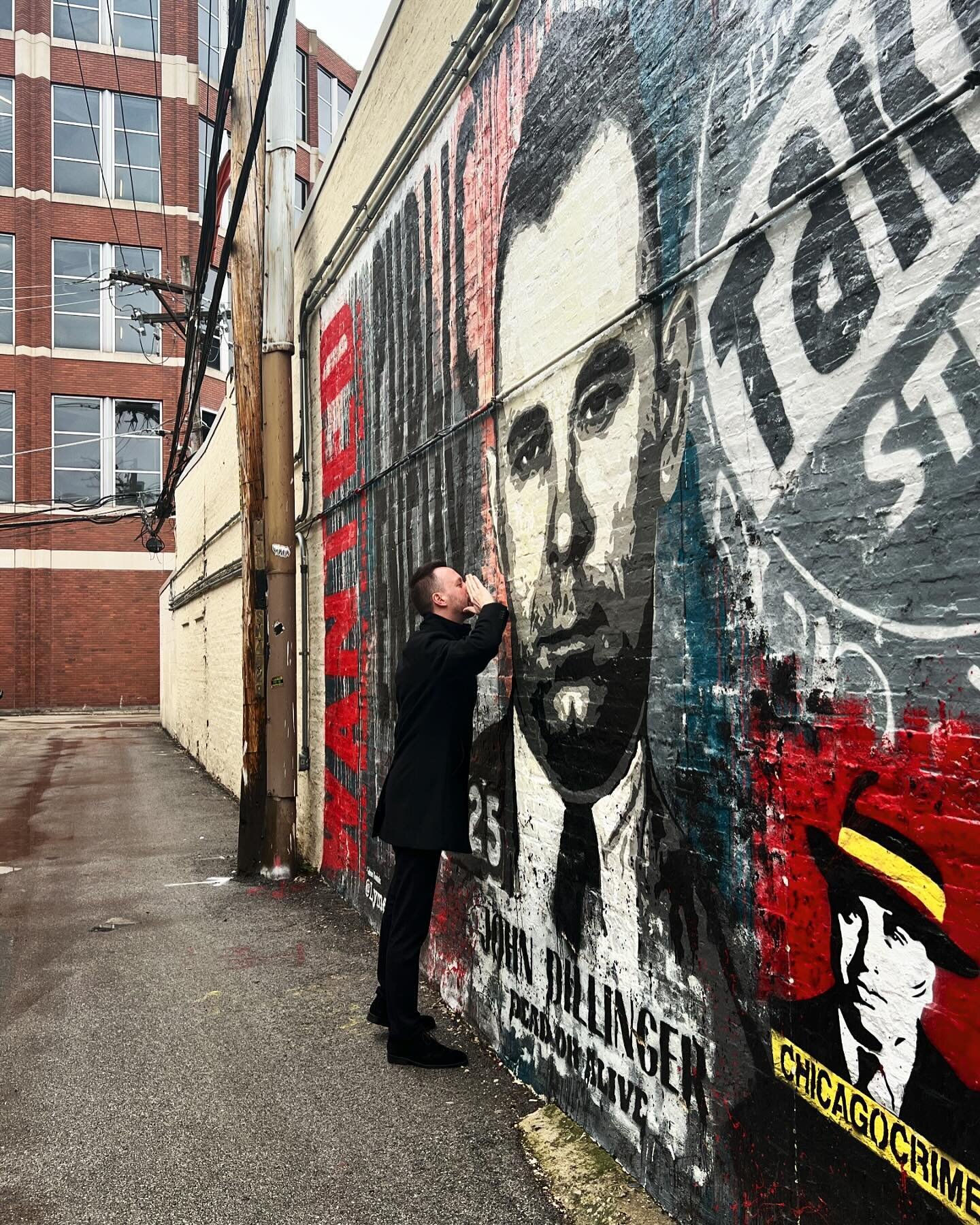In the image, a man stands in a wet city alleyway, whispering into a large wall mural of John Dillinger, a notorious gangster from the 1920s United States. The mural, predominantly in blacks and whites with touches of red, features a bold portrayal of Dillinger, with a smaller depiction of Al Capone, labeled “Chicago Crime” in the lower right corner. The man, dressed in an all-black suit, mimics speaking a secret into Dillinger’s ear, creating a humorous juxtaposition against the serious historical context of the murals. The scene is further detailed by the wet alleyway, suggesting recent rain, and a brick building towering in the background. The vibrant, multicolored wall adds a striking contrast to the otherwise somber tones of the mural and the surrounding urban landscape.